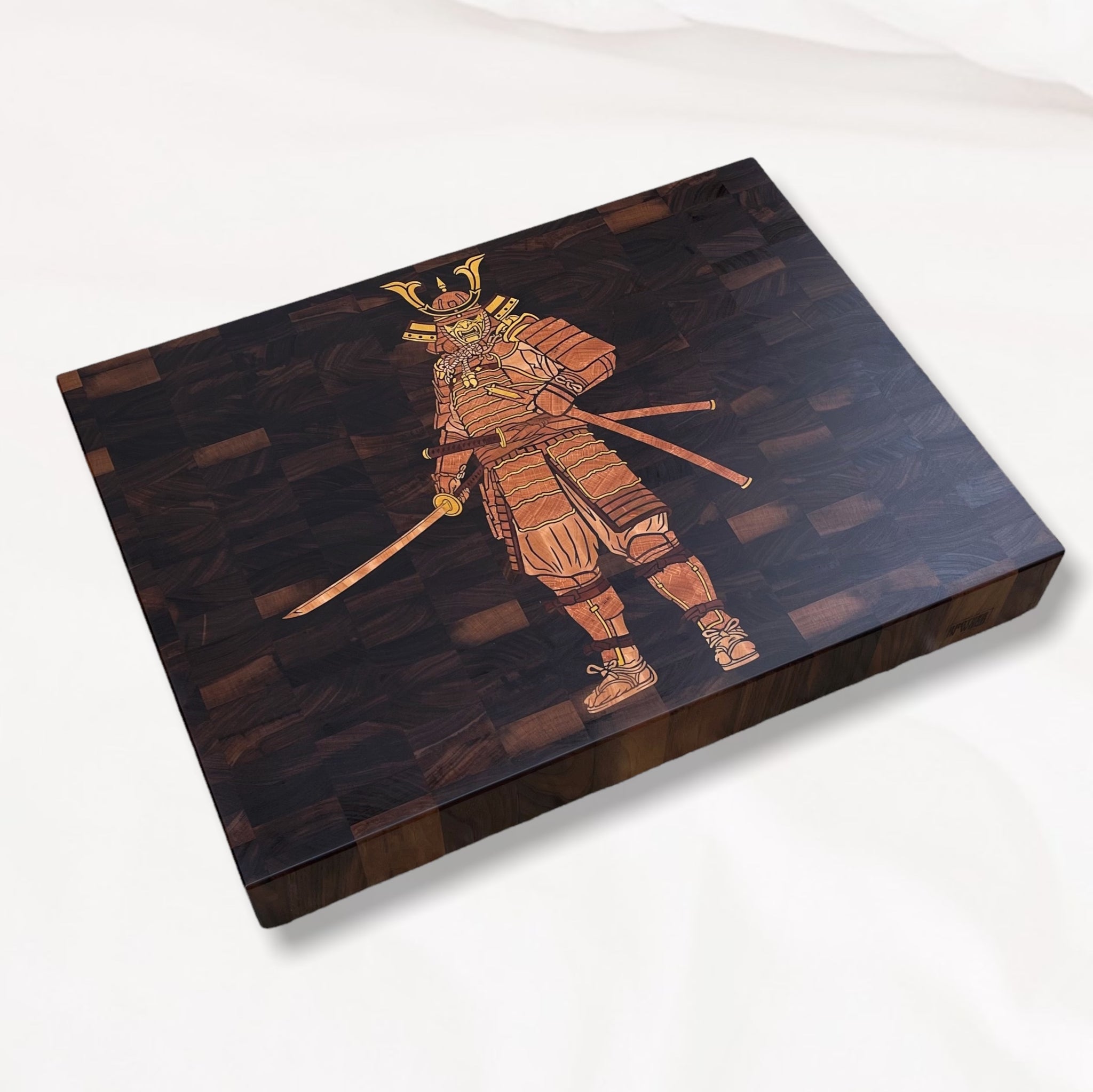The image depicts a detailed illustration of a Japanese samurai warrior, rendered in shades of orange, gold, and black, on a wooden parquet block with both dark and light pieces. The block is placed on a white background and is slightly rectangular. The illustration shows the samurai standing in a battle-ready pose, holding a katana in his right hand and its sheath in his left hand, with an additional sword attached to his waist. The warrior is adorned in heavy armor that protects his body, legs, shoulders, and shins, and he is wearing traditional sandals tied around his ankles. His fearsome mask, with fangs and a grimacing face, is partially covered by a helmet featuring a U-shaped piece of metal and a spike on the dome, emphasizing his readiness for combat. The background of the illustration appears brown, resembling marble or rubrics, and the entire painting is positioned diagonally, adding a dynamic angle to the composition.